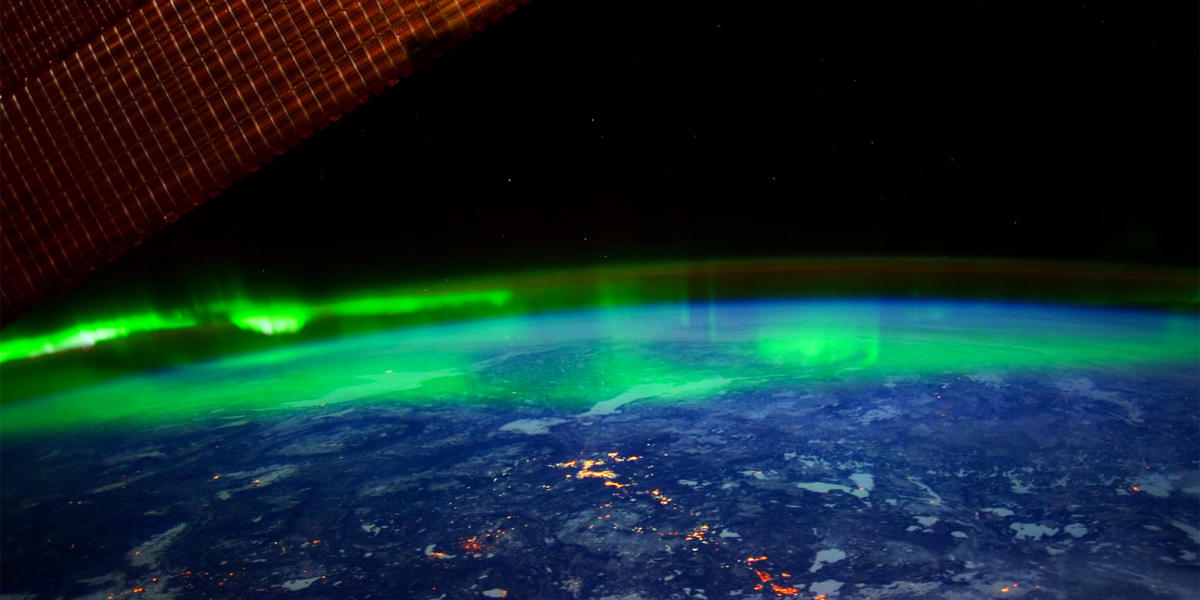This vibrant and detailed image, appearing to be captured from outer space, showcases a striking top-down view of a planet or Earth. The greyish-blue surface of the land is prominently cut through by a glowing, molten lava-like river, creating a dramatic contrast. Encircling the planet at its outer rim are stunning green northern lights, evoking the Aurora Borealis. In the upper left corner of the image, a satellite-like grid structure, colored reddish-orange, adds another layer of intrigue with its segmented squares and a narrow diagonal board. The backdrop of the night sky enhances the otherworldly ambiance, making this scene reminiscent of a sci-fi movie or an AI-generated artwork. The overall setting is unmistakably in space, highlighting the beauty and mystery of the cosmos.